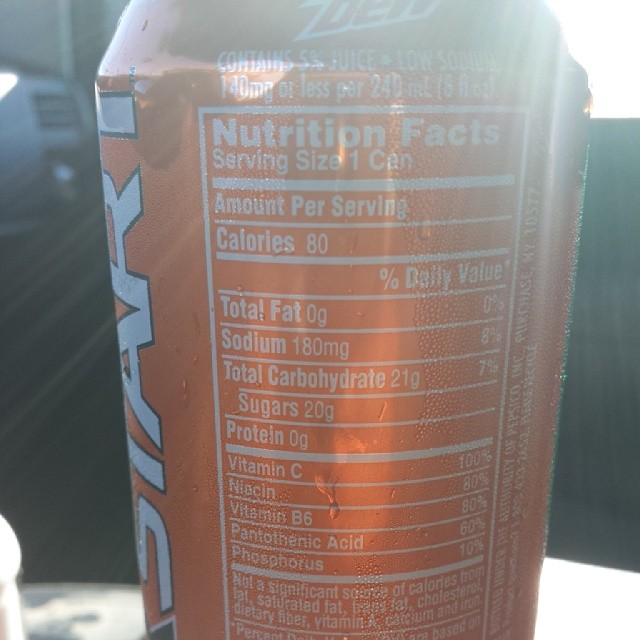This close-up photograph showcases the side of an orange can, likely a Mountain Dew Kickstart, featuring detailed nutritional information. The can is adorned with hard-to-read white lettering spelling "START" partially visible along with a small black symbol outlined in white. The label prominently displays nutritional facts within a white graph, listing: 80 calories, 0g total fat, 180mg sodium, 21g total carbohydrates, 20g sugars, and 0g protein per serving (1 can). The drink contains 5% juice and boasts 100% daily value of Vitamin C, 80% of Niacin and Vitamin B6, and 60% Pantothenic acid, with 10% phosphorus. The surface of the can glistens with condensation, hinting at its cold refreshing contents. There is a glare in the photo, suggesting it was taken in a brightly lit environment, potentially in a car given an indistinct vent-like shape in the background.